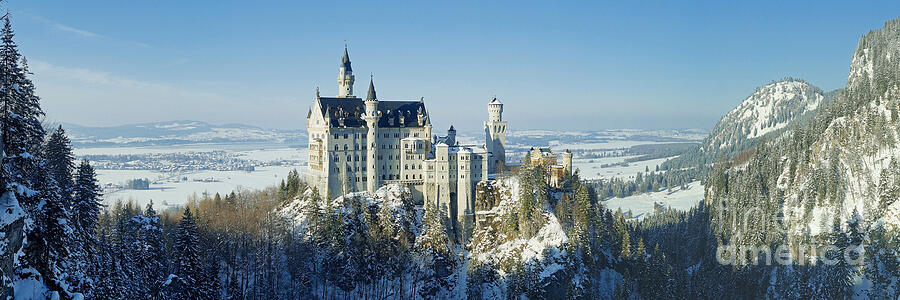In this panoramic photo captured from a great distance, a grand, fairytale-like castle stands majestically atop a rugged mountain precipice. The castle, reminiscent of historical structures found in Germany, is predominantly white with a striking blue roof and features multiple turrets, topped with pointy ends. Dominating the landscape, the castle is a complex edifice of four to five stories, with interconnected structures and towers contributing to its grandeur.

The scene is set in a winter wonderland, with snow blanketing the landscape and scattered across the valley that extends to a plain below. Evergreen trees dot the left side, while to the right, rugged mountains and large hills rise, creating a dramatic backdrop. The setting under clear blue skies enhances the serene and magical atmosphere. The bottom right corner of the photo includes a delicate caption in thin, lowercase letters reading "fine art America," suggesting its artistic value.